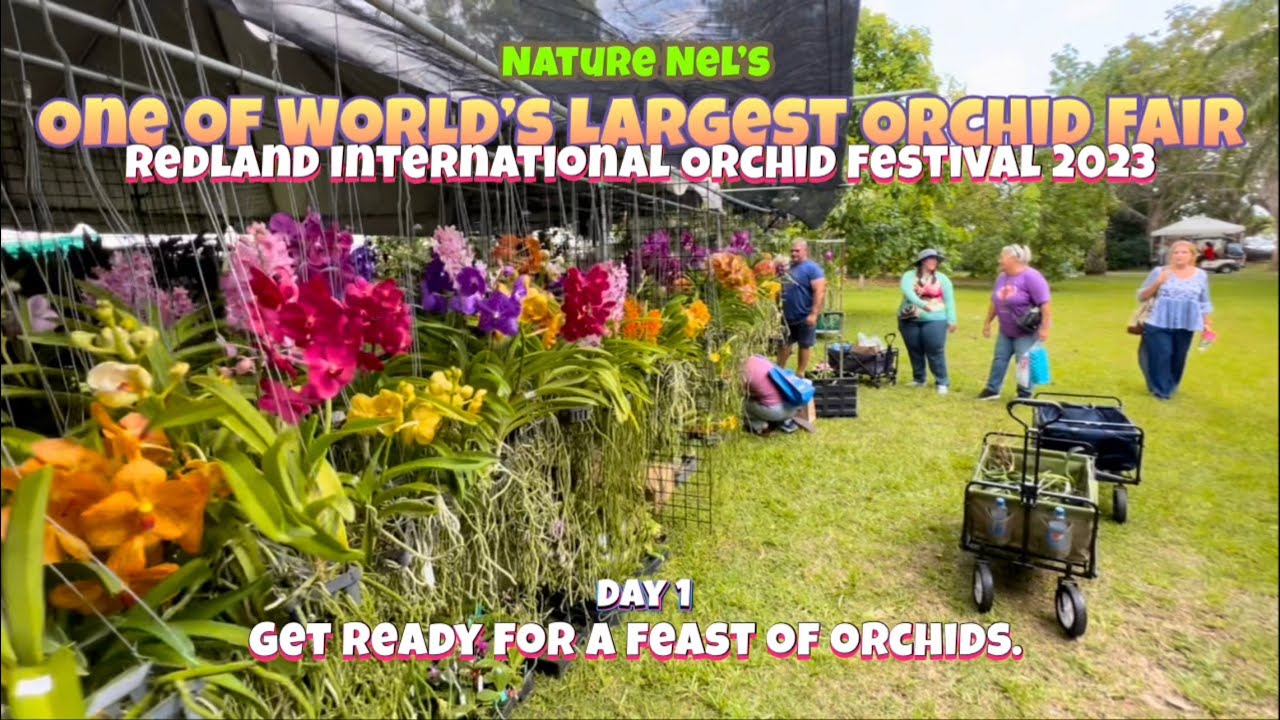This rectangular outdoor promotional photograph, approximately six inches wide by three inches high, depicts the vibrant atmosphere of the Redland International Orchid Festival 2023. The top of the image features bold text in light green, reading "Nature Nills," followed by light peach text with a purple outline announcing "One of the World's Largest Orchid Fairs." Further down, white text with a red outline proclaims "Redland International Orchid Festival 2023." 

The bottom of the image features white text with a blue outline stating "Day One," and directly below, white text with a red outline encourages "Get Ready for a Feast of Orchids."

In the foreground, on the left side, rows of multi-colored orchids—orange, pink, yellow, purple, and white—are displayed as if hanging from baskets or arranged on tall stalks. These flowers stretch back towards a black-tented area, creating a stunning floral display. Among the blooms, five people, dressed in gardening attire including jeans, are either standing or kneeling, tending to the plants. Some are working with carts or four-wheeled wagons filled with gardening accessories that may include weeds.

Towards the right side of the image is a grassy area with people in gardening clothes moving about. In the far background, trees frame the scene, adding a natural border, while a red-shirted person sits under an umbrella, partially hidden by the vibrant activity.

Overall, this promotional image captures the anticipation and excitement of the event, with its lush array of orchids and busy, diligent gardeners set against a picturesque outdoor backdrop.